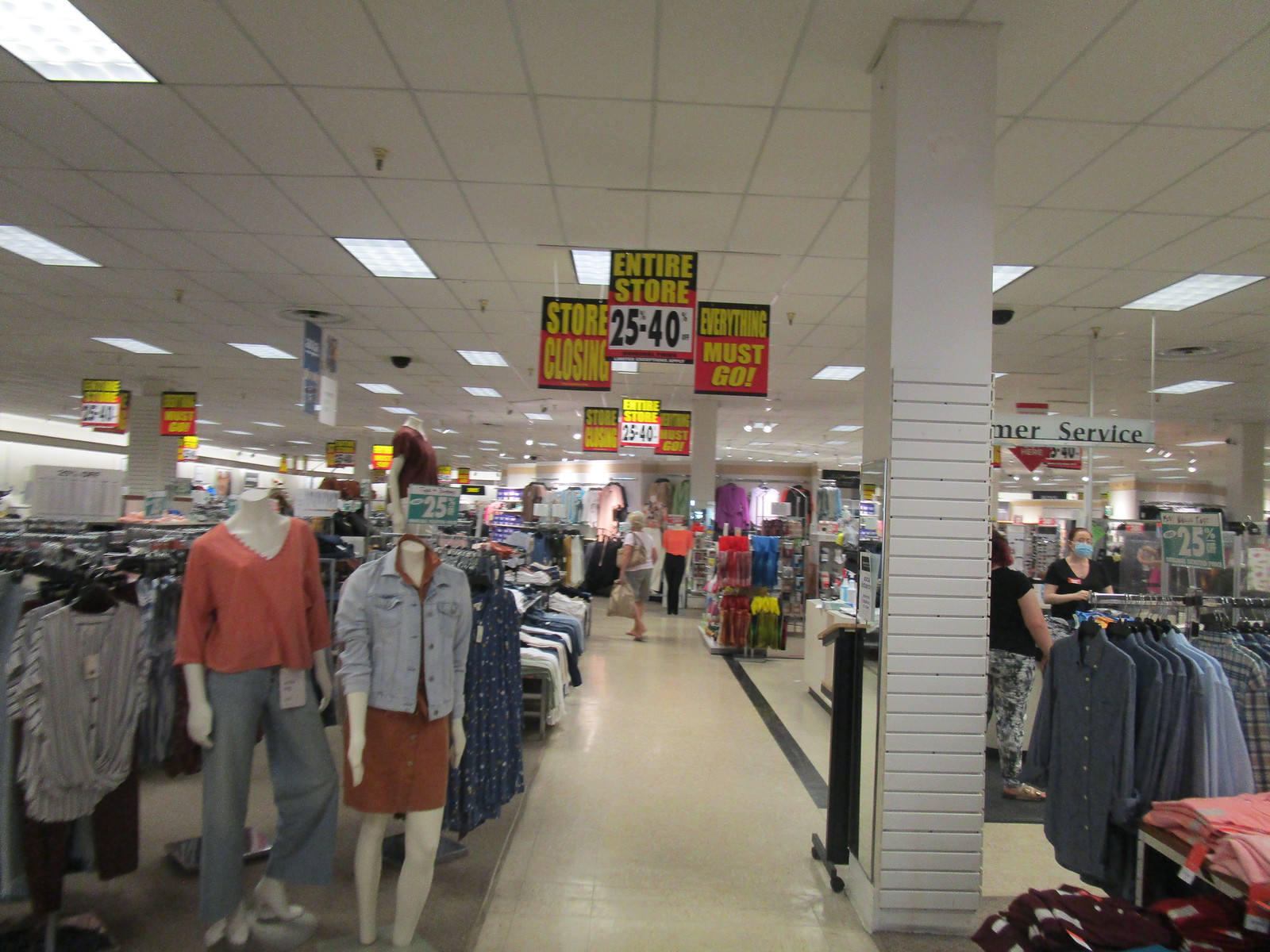This is a photograph taken inside a nondescript department store, possibly one like Sears or J.C. Penney, during the pandemic. The store appears mid-range, not high-end, and features a grid of acoustic tiles on the ceiling with recessed fluorescent lights. Some white pillars rise up into the ceiling. The floor is tiled in beige with black border tiles separating different sections for products.

We see a walkway leading deeper into the store, lined on the left with various women's clothing items such as shirts and pants, and on the right with men's shirts and more women's clothing. Prominently displayed are two mannequins: one wearing a pink or salmon-colored top with three-quarter-length sleeves and wide flare-out pants or jeans, and the other dressed in a denim jacket with a brown dress. Another mannequin is dressed in loose-fitting boyfriend jeans and a v-neck top.

Hanging from the ceiling are numerous signs in black, red, and yellow that read "Store Closing," "Entire Store 25 to 40% off," and "Everything Must Go." These signs repeat down the aisles, emphasizing the store's closing sale. The customer service sign is visible behind a column on the right side. Several shoppers mill about, including one woman in a blue face mask and another woman holding a purse and examining merchandise. An employee, noticeable by her name tag and light blue surgical mask, involved in what seems to be part of the store’s operations, further indicates this scene is from the pandemic period.